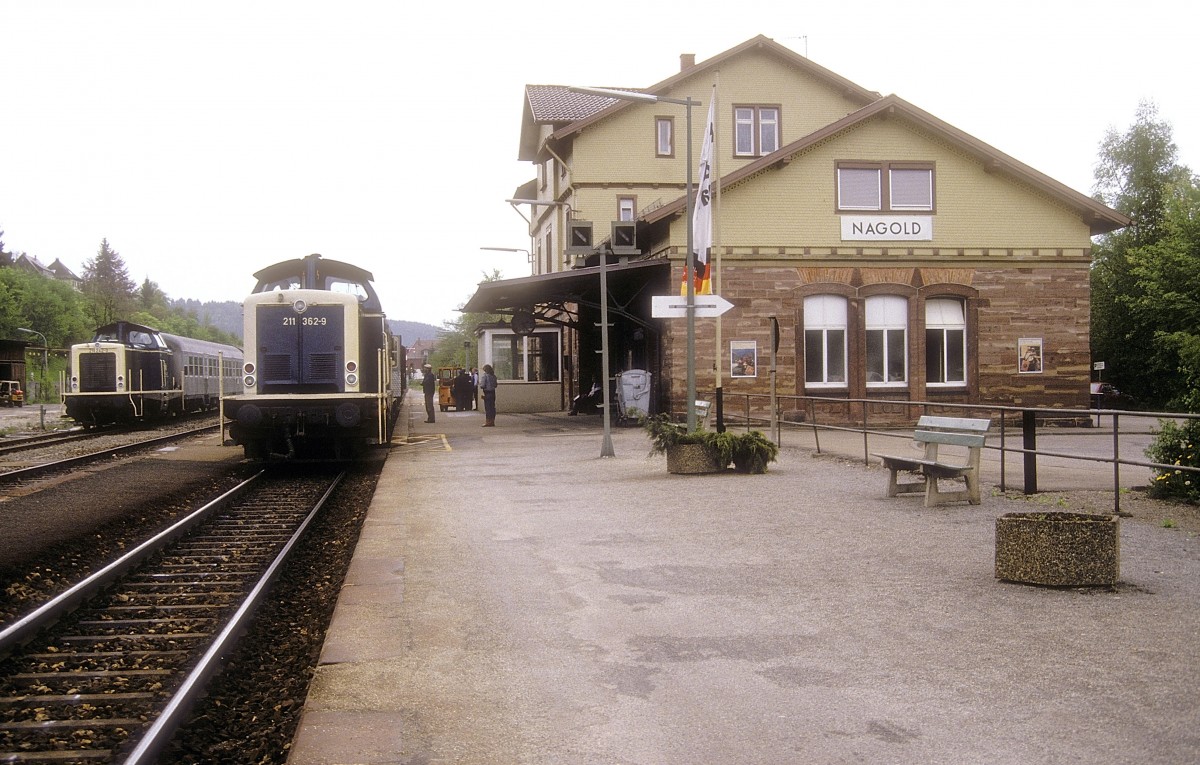This detailed photograph depicts a bustling train station, likely situated in Germany. On the left side of the image, two substantial trains, painted in navy blue with white stripes, are stationed on their respective railroad tracks. The forefront of these trains faces the viewer. Adjacent to the tracks, lush trees and rooftops are visible, with hills faintly discernible in the distant background.

Dominating the center to the right side of the photograph is the train station's structure and surrounding area. The station itself is a three-story building, with the lower portion constructed from sturdy brown stone, containing several windows. The upper portion is made of tan and cream-colored wood siding, adorned with numerous windows and an angled roof reminiscent of a traditional house. “NAGOLD” is prominently displayed in capital letters beneath the windows of the building. A white flag flutters on a flagpole near the station.

The platform and surrounding area, dotted with circular planters, benches, and a few waiting passengers facing the trains, provide a glimpse into daily life at the station. The scene is one of serene anticipation amidst the architectural blend of stone and wood, with natural elements framing the station in a picturesque setting.